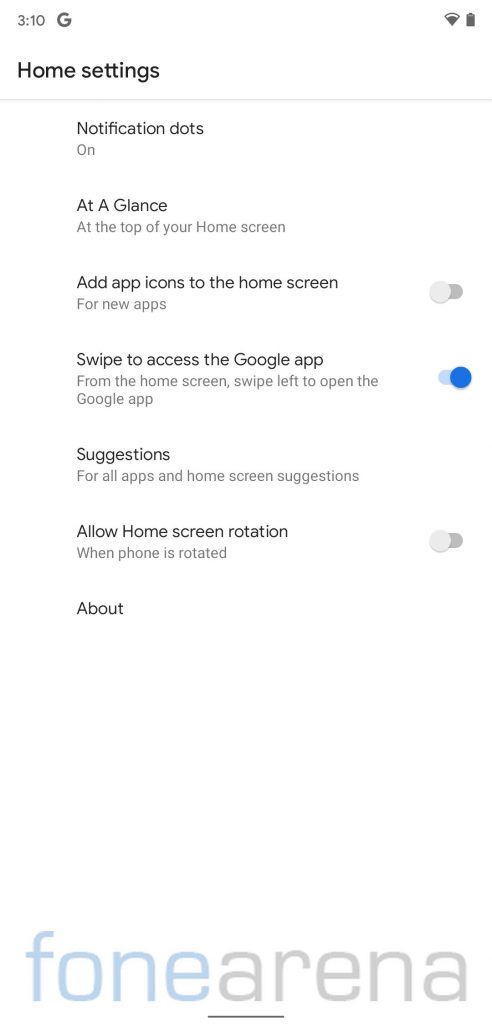A screenshot of a website displayed on a mobile phone shows the interface of "FONE Arena," with "FONE" prominently colored in blue and "Arena" in a tan-grayish hue. At the top right corner of the screen, indicators display cellular connection strength and battery life, while the top left shows a "G" and the time, 3:10. Below the top bar are black text options for "Home" and "Settings."

Several settings are displayed under a header bar which reads "Notification dots on," indicating they are enabled. Further options describe various settings for the home screen: "At a glance at the top of your home screen" and "Add app icons to the home screen for new apps" (which is turned off and grayed out). The option to "Swipe to access the Google app" is turned on, with instructions to swipe left from the home screen. Additionally, there are settings for "Suggestions for all apps and home screen suggestions," and an "Allow home screen rotation" toggle that is turned off, noting that it applies "when phone is rotated."

Near the bottom of the screen, the word "About" appears, but there is no accompanying text. The background of the website is white, and at the very bottom, "FONE Arena" is repeated, with a line under the "A" in "Arena."